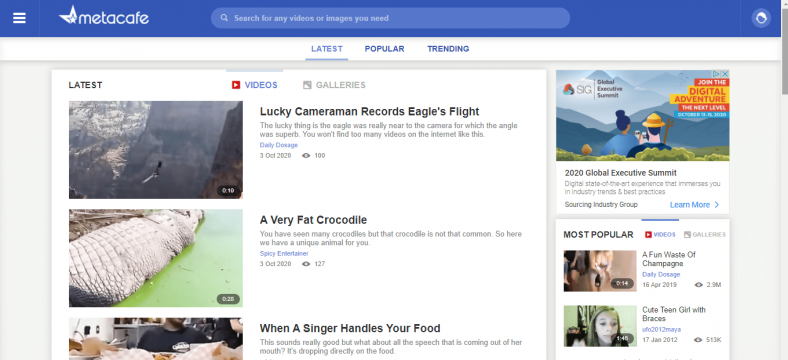The Metacafe website features a predominantly blue and white theme. At the top, a blue rectangular bar houses a three-line menu icon beside the Metacafe logo, followed by a search bar. Beneath this, there are blue tabs labeled "Latest," "Popular," and "Trending." Below these tabs, and set against a white background, the main content area begins with the section labeled "Latest," which is then subdivided into sections titled "Videos" and "Galleries."

The "Latest" section showcases three video thumbnails. The first caption reads, "Lucky camera records eagle flight," and the corresponding image appears to be an aerial shot of mountains. The second caption, "A very fat crocodile," features a thumbnail of a notably large crocodile. The third caption, "When a singer handles your food," includes an image hinting at a singer possibly involved in a restaurant setting, although the details are not clearly visible.

To the right of these video thumbnails, there is information about the "2020 Global Executive Summit," which includes links to related videos. Below this, in the "Most Popular" section, the first video listed is titled "A fun view of Champagne," followed by another video named "Cute Teen Girl with Braces."